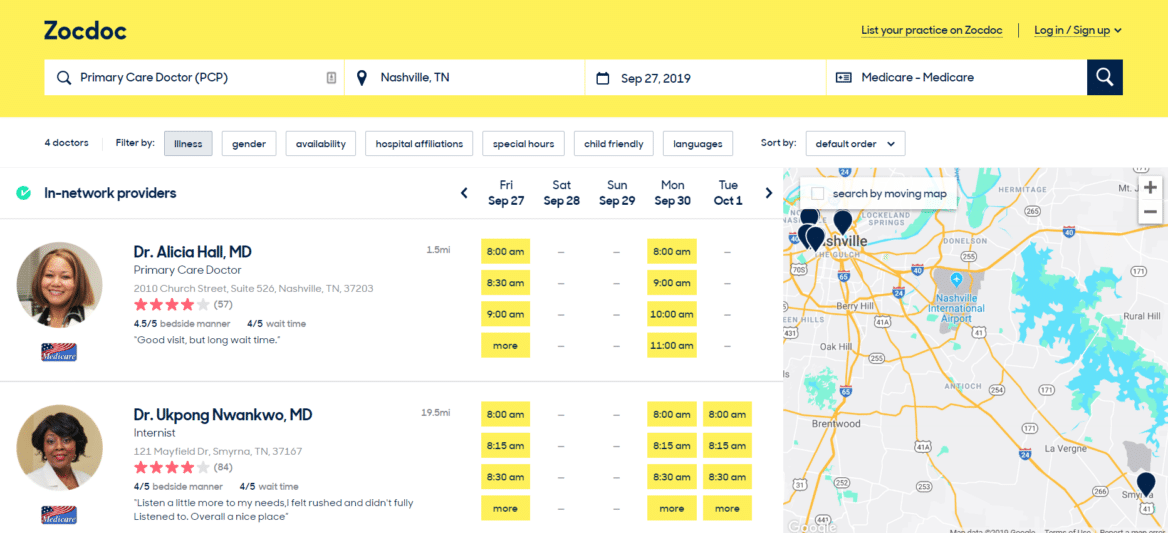The image is a detailed screenshot from the ZocDoc website, showcasing a search interface for finding doctors in Nashville, TN.

In the upper left corner, the ZocDoc logo is displayed in black letters within a long yellow box. Just below the logo, there's an interactive yellow search bar containing a long white box where users can enter different search options. The search options include "Primary Care," "Select Doctor," and "PCP" in black text. To the right of these options, "Nashville, TN" is displayed next to a location icon followed by a calendar icon showing the date "Sep 27, 2019." Further to the right, there is an icon resembling a square with several horizontal lines, labeled "Medicare/Medicaid." A black square with a white magnifying glass icon is positioned at the search bar's end.

Above this search bar, the phrase "List your practice in ZocDoc" is underlined in black, offering a clickable link. Below, there's a faint gray line with an option to "Login/Sign up" underlined, accompanied by a downward-pointing black V.

The main body of the screenshot features a filter section. From left to right, the filters are highlighted in gray and include options such as "Illness," "Gender," "Availability," "Hospital Affiliations," "Special Hours," and "Child-friendly Languages." There is also a "Sort by" option in black text, followed by a downward-facing V.

To the right, a prominent aqua-colored circle with a white checkmark denotes "In-network providers." This section also features several dates indicated between sideways-facing Vs, suggesting navigation through available appointment dates. The top row lists "Fri, Sat," "Sun," "Mon," followed by calendar dates "Sep 27," "Sep 28," "Sep 29," "Sep 30," and "Oct 1."

Displayed below the filters are profile snippets of two doctors. The first profile shows a circular photo of Dr. Alicia Hall, a Caucasian woman with short brown hair, wearing a white lab coat against a gray background. Her profile indicates she is a Primary Care Doctor in Nashville, with a rating of 4 out of 5 stars from 57 reviews. The reviews highlight her bedside manner and wait times, summarized as "Good visit but long wait time." Available appointment times are listed in yellow boxes with black text.

The second doctor is Dr. Ukpong Ngwango, whose profile features a circular photo of an African American woman with short black hair in a white lab coat, set against a tan background. She is an Internist located in Smyrna, TN, with a rating of 4 out of 5 stars from 84 reviews. The review mentions feeling rushed but overall describes the clinic as "a nice place." Her available appointments are also shown in yellow boxes with black text.

To the right of the doctor profiles, there is a map of southeastern Nashville displaying the locations of the various doctors with blue pins.